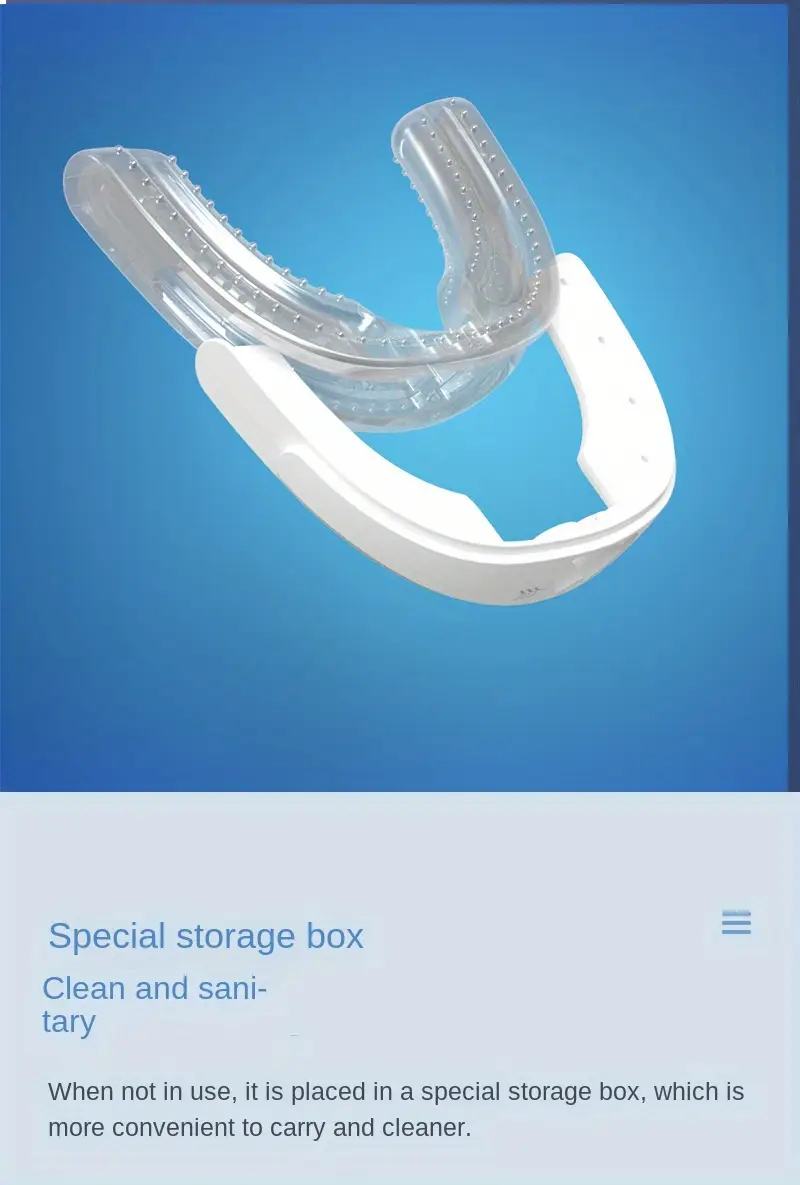The image is a horizontally aligned rectangle divided into two sections. The upper section features a solid blue background showcasing a clear plastic retainer, positioned as if ready to fit into a white storage case beneath it. This background provides strong contrast, clearly highlighting the retainer and its accompanying storage case. The lower section is a light gray rectangular box that contains text. In the upper left corner of the gray section, blue text reads "Special storage box, clean and sanitary." Below, in black text, it states, "When not in use, it is placed in a special storage box which is more convenient to carry and cleaner." The image is bright and clear, with no other objects present, making it easy to see and understand. The setting emphasizes the retainer and storage box, suggesting a product for sale aimed at promoting cleanliness and convenience.